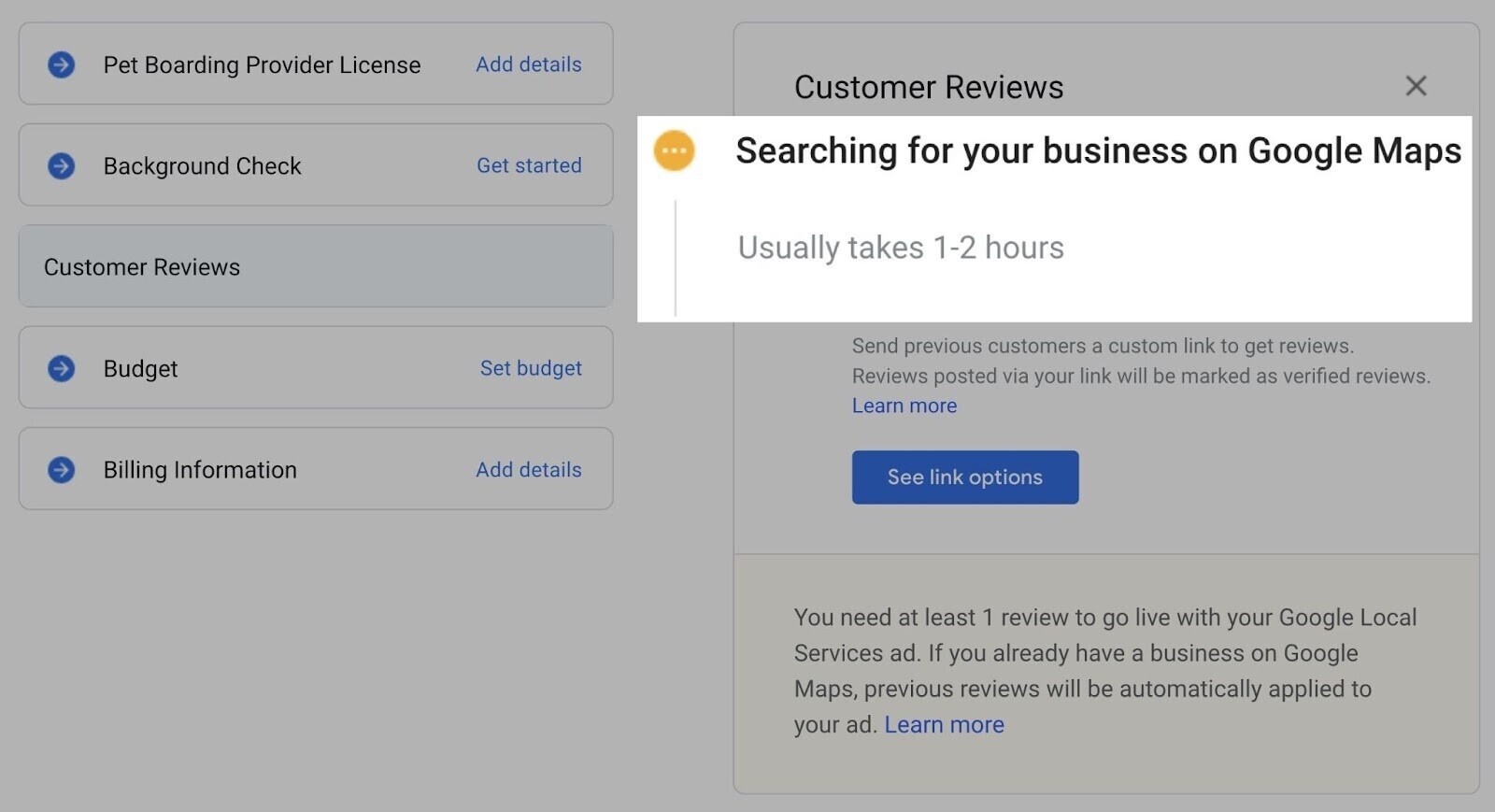This image is a screenshot of a webpage, displayed in a grayed-out state, with a prominent white pop-up in the foreground. The pop-up features a yellow circle on the left containing three vertical white dots. The pop-up's main message is written in bold black text stating, "Searching for your business on Google Maps," with a subtext in gray noting, "Usually takes one to two hours."

In the background, the grayed-out website includes a navigational menu on the left side. This menu features categories such as "Pet Border Provider License Background Check," each accompanied by blue circles and right-pointing arrows. Below these categories, there is an "Add Details" button and a "Get Started" call-to-action button.

Further down the grayed-out page, a slightly darker section is labeled "Customer Reviews" prominently. Below this, additional blue-circled options like "Set Budget" and "Billing Information" are listed, each with arrows pointing to the right. The "Customer Reviews" section also includes detailed information explaining how to send previous customers a custom link to gather verified reviews, marked distinctly by an “X” on the right. 

Messages below explain that "You need at least one review to go live with your Google Local Services Ad. If you already have a business on Google Maps, previous reviews will automatically be applied to your ad." This section includes a "Learn More" button and a "See Link Options" button in a blue rectangle for further action.